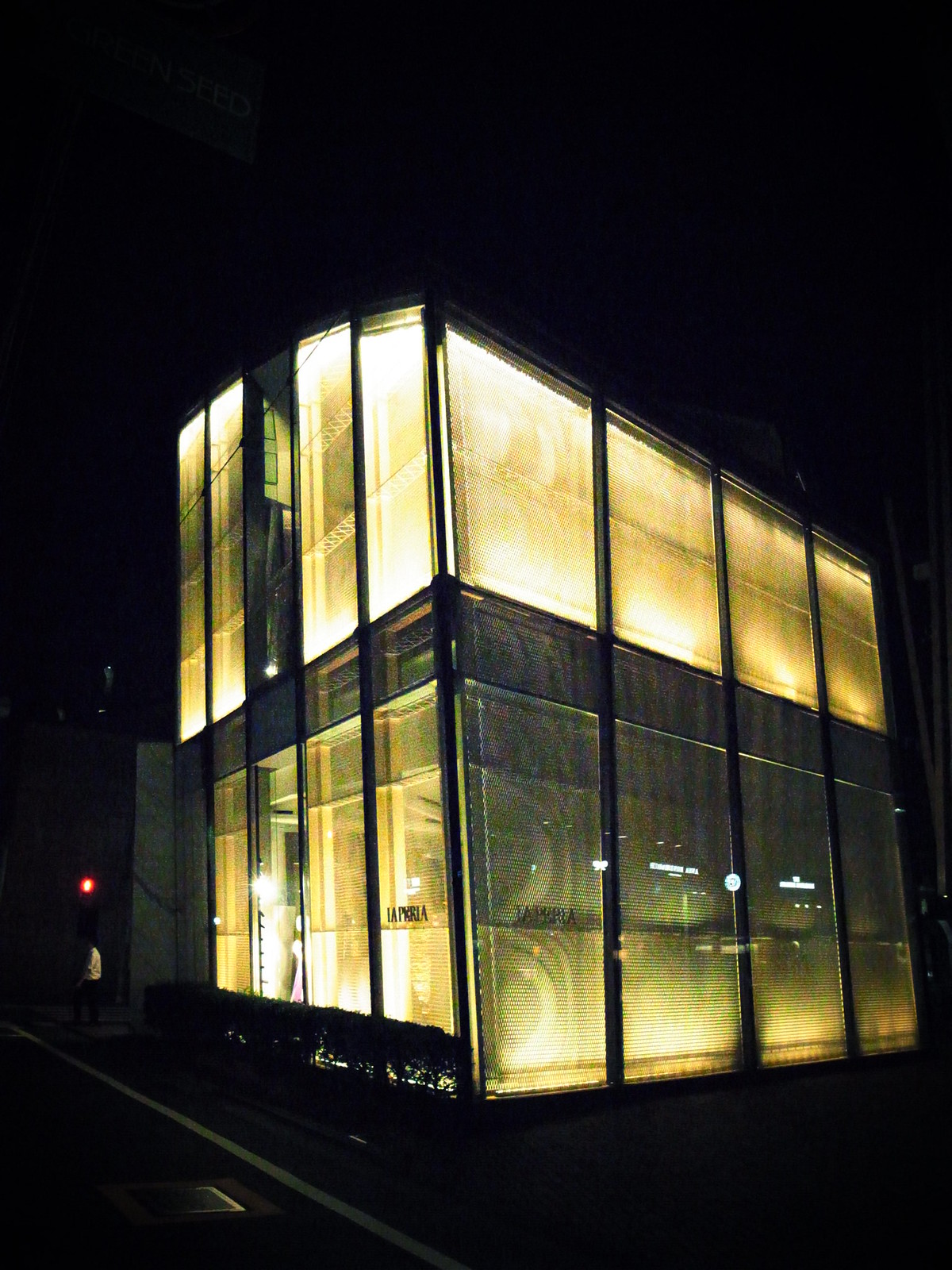The photograph captures a striking two-story building entirely wrapped in floor-to-ceiling glass panels, framed in metal. Set against a pitch-black night sky, the structure glows from within, with almost all indoor lights turned on, casting a warm yellow hue. The building's transparency is interrupted by gray fabric curtains pulled down, preventing a clear view of the interior. The ground level showcases a neatly landscaped hedge near the entrance, while the left bottom corner foreground displays an asphalt road with an angled curve and a water drainage grill. Additional urban elements include the faint outline of a car, a red stop sign in the distance, and a pedestrian standing near a red light at what appears to be an intersection. Text on the glass panels reads "La Perio," adding a hint of commercial identity to the luminous, glass-box-like structure.